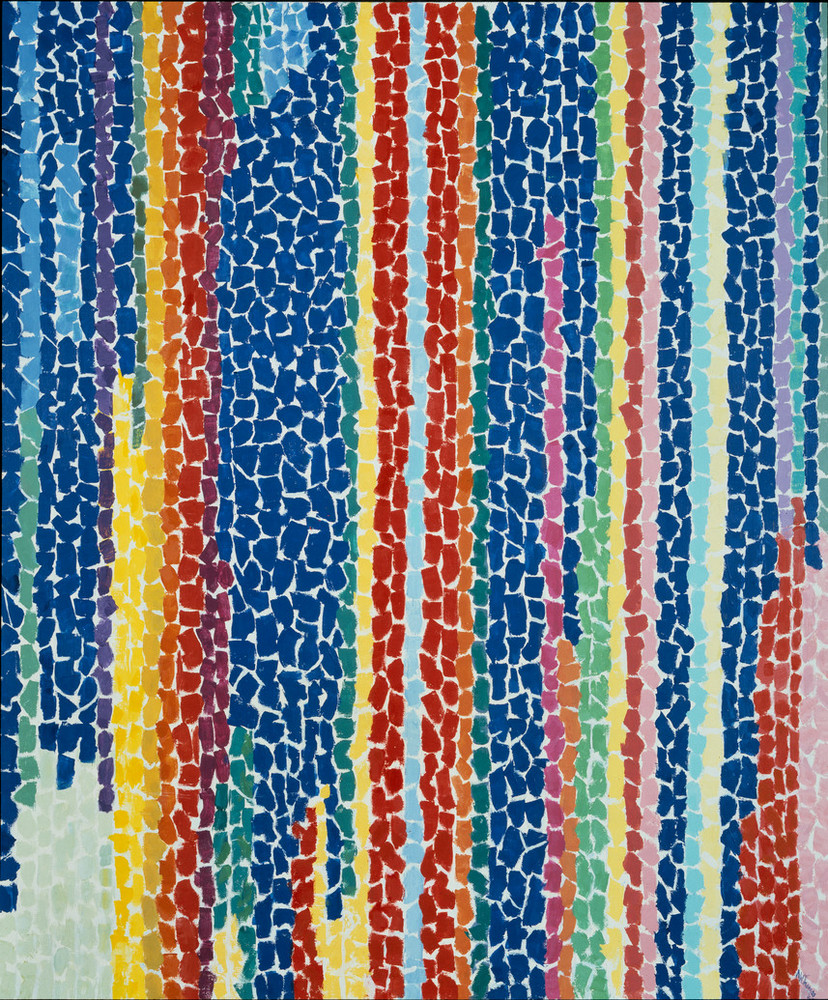This painting is an intricate abstract work displaying a series of vertical lines made up of jagged, mismatched shapes, creating an appearance of tiles. Dominated primarily by dark blue hues, the painting incorporates a rich palette of colors including light green, light blue, yellow, muted yellow, gold, orange, burnt orange, red, pink, purple, and white. Each line, comprised of different colored segments, runs from top to bottom, contributing to the dynamic and colorful pattern that spans the slightly rectangular, portrait-oriented canvas. The artwork is bordered by a thin black line, framing the visually complex and vibrant display.